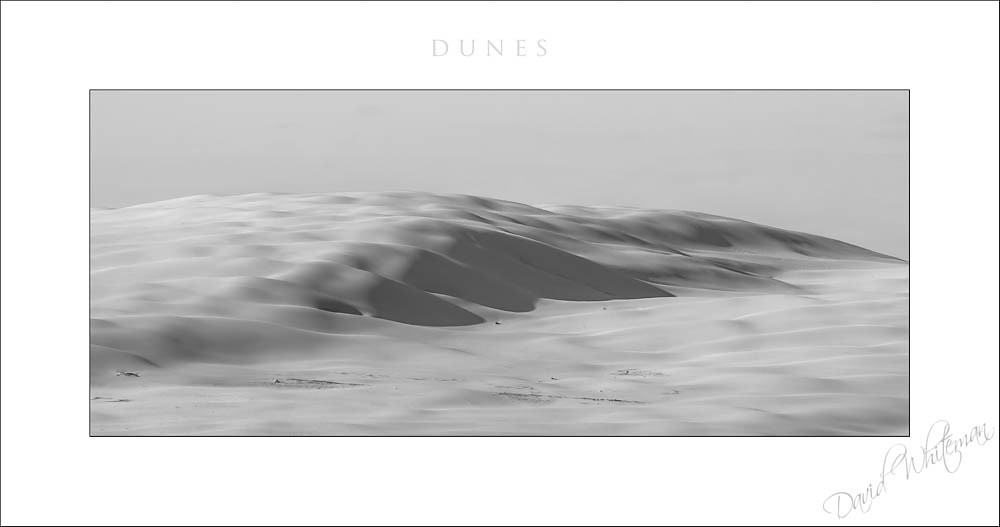The image is titled "Dunes" and features vast, undulating sand dunes extending to the skyline, creating a tranquil and smooth visual effect. The photograph, primarily in shades of white and gray, captures the ethereal beauty of the landscape under a gray sky. Lighter shades of white and light gray highlight the dune crests, while darker gray tones accentuate the lower elevations and ripples of the sand, reminiscent of water. Encased in a white border, the photograph exudes a timeless quality. At the bottom right-hand corner, the artist's signature, 'David Whitman', graces the image, adding an element of authenticity.